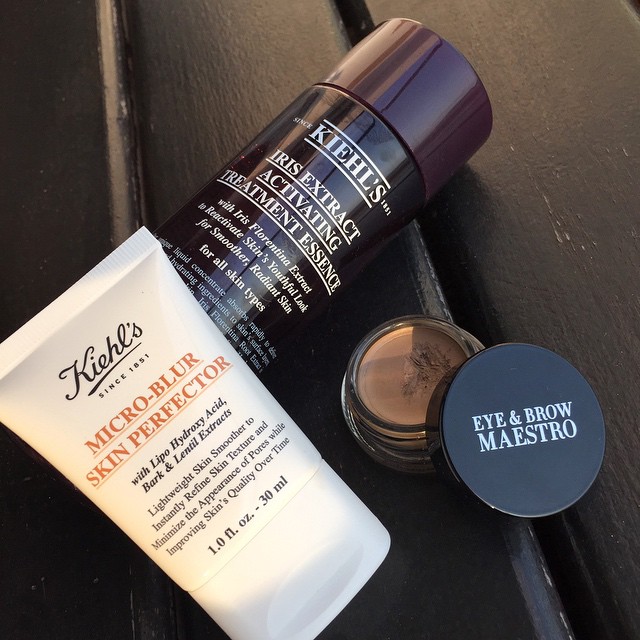The image features a collection of skincare products neatly arranged on a black-painted wooden bench. In the bottom left, there's a white plastic tube labeled "Kiehl's Since 1851 Micro Blur Skin Perfector," and beneath it, the text mentions ingredients such as lipo-hydroxy acid, bark, and lentil extracts, with a volume of 1 fluid ounce (30 milliliters). To its right, there's an opened glass container with a black lid labeled "Eye and Brow Maestro." This container of brown eyebrow cream has been visibly used, with a noticeable indentation where some product has been taken out. Finally, at the top left, there is a cylindrical black bottle with a matching black cap, inscribed with "Kiehl's Iris Extract Activating Treatment Essence," highlighting the use of Iris Florentina extracts to promote a youthful, radiant complexion suitable for all skin types. The products are thoughtfully laid out, showcasing a mix of skincare and makeup essentials.